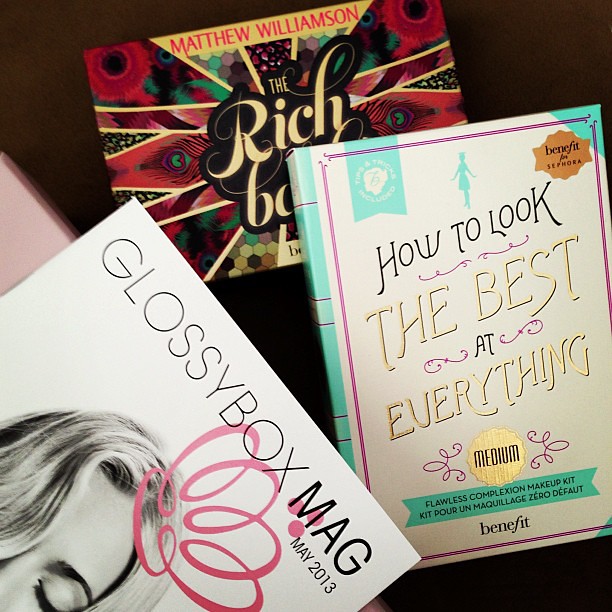This image features a dark background with a variety of items partly truncated, including books, a magazine, and a makeup kit. In the lower left, there is a white magazine titled "Glassy Box Mag, May 2013." It displays the top part of a woman's head with closed eyes and a pink tiara drawn in. To the right of the magazine is a cream-colored box with green accents labeled "How to Look the Best at Everything: Medium Flawless Complexion Makeup Kit" by Benefit. Behind this makeup kit, there appears to be a postcard or packaging with a vivid design that incorporates red, black, and green peacock feathers and gold lines radiating from gold text. The visible text reads "Matthew Williamson" in red on a yellow background at the top, and "The Rich" partially obscured by the makeup kit.